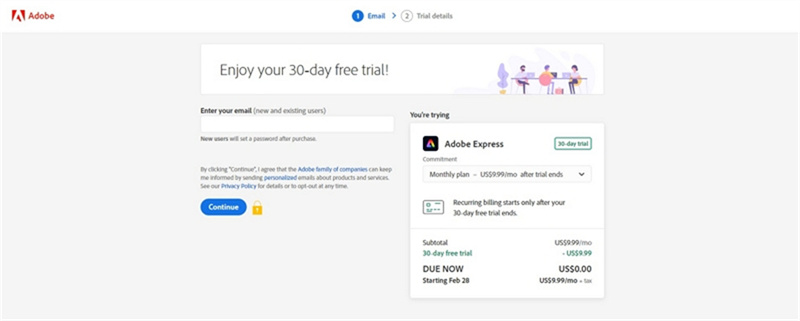A screenshot of the Adobe website features prominently in this image. The page confirms that an individual has just signed up for a 30-day free trial of Adobe Express starting on February 28th. The background is a neutral gray, with a bold message stating, "Enjoy your 30-day free trial." 

The page requests the individual to enter their email address, which remains incomplete. Additionally, there is a comprehensive breakdown of the trial details, indicating that no charges will be applied during this period. 

The screenshot also includes a section presenting Adobe's privacy policy, ensuring the user understands how their data may be used and shared, in compliance with federal agency regulations. Although the text in the screenshot is quite small and difficult to read, the overall layout and essential information convey a clear message about the trial subscription and privacy disclosures.